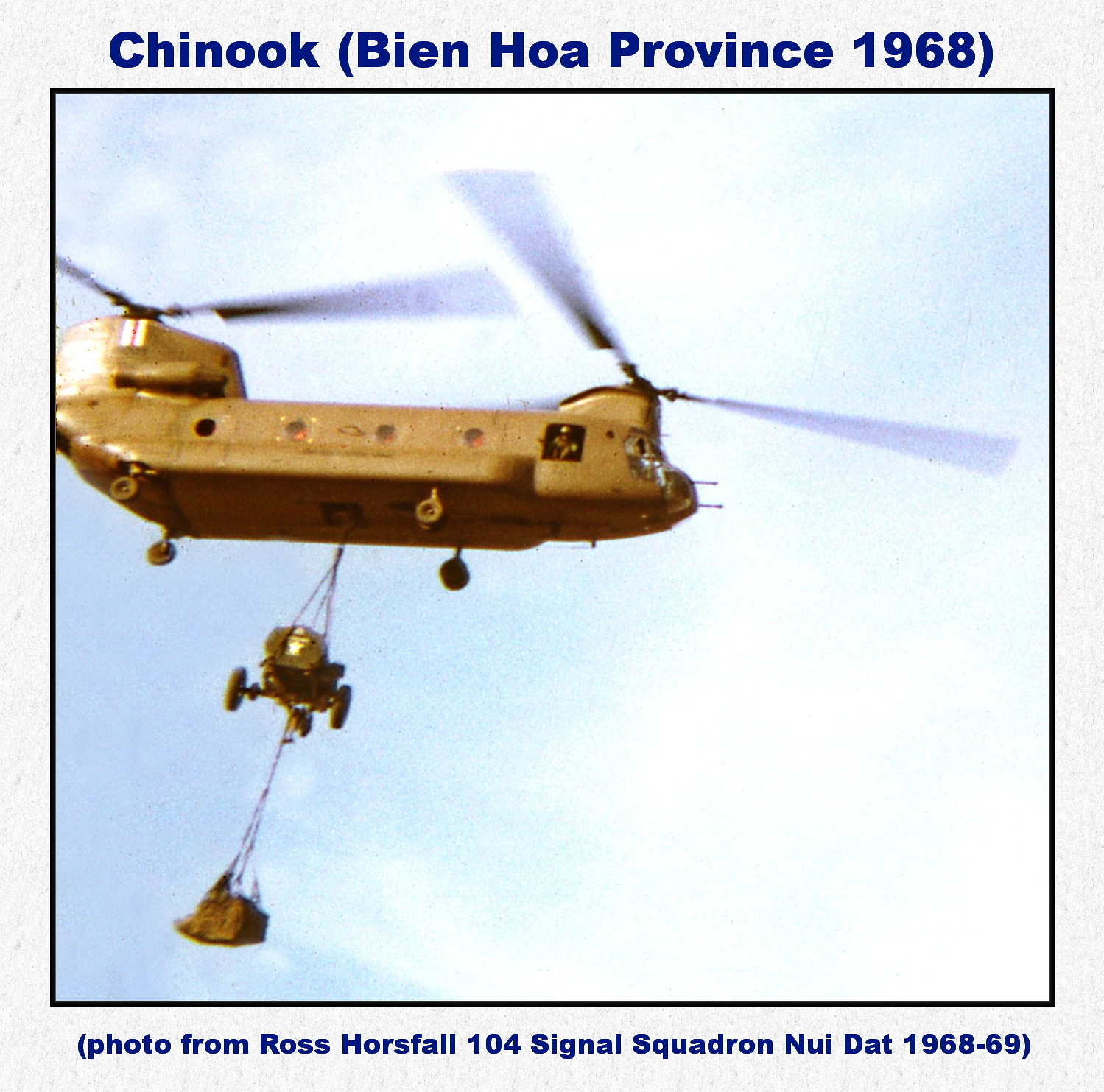The image depicts a dual-rotor military helicopter, identified as a Chinook, against a light blue and white cloudy sky, suggesting it is midday and outdoors. The background features an off-white textured border, framed by a black line. The helicopter is painted in a brownish-green color, typical of military camo, with distinctive vertical white and red stripes at one end. It has antennas protruding from the nose, four visible windows along its fuselage, and is equipped with four landing wheels. The Chinook, with rotors positioned at both the front and back, is carrying a payload: an artillery piece mounted on wheels, suspended by chains from its midsection, and a crate-like object wrapped in sturdy material hanging below that. Moreover, you can catch a glimpse of a person through one of the open side doors. The text overlay at the top of the photograph reads, "Chinook, Bien Hoa Province, 1968," pinpointing the location to Vietnam during the early Vietnam War period. A photo credit at the bottom states, "Photo from Ross Horsfall, 104 Signal Squadron, Nui Dat 1968-69."